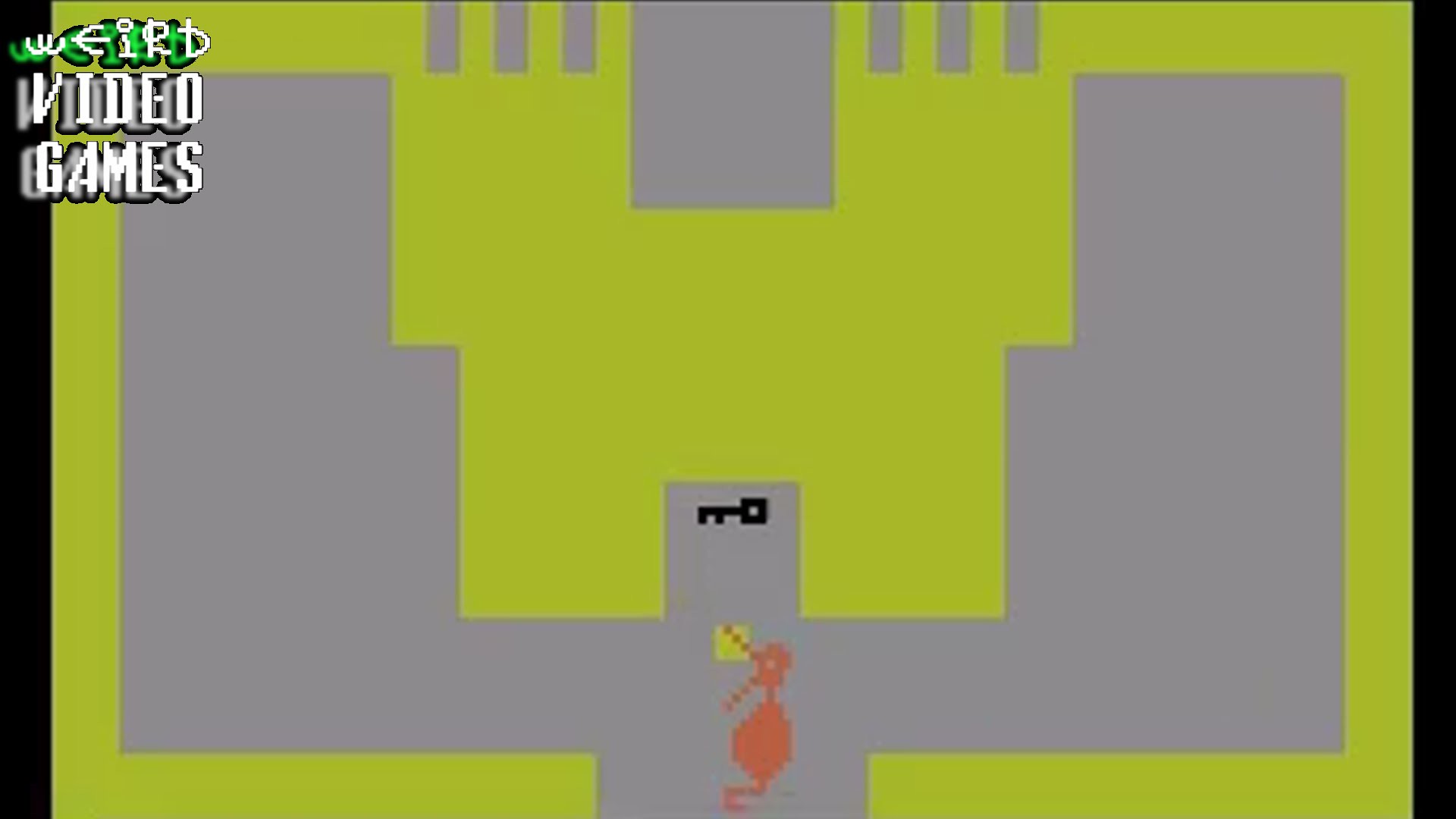The image showcases a video game screen framed with black borders on both the left and right sides. In the upper left corner, "Weird Video Games" is prominently displayed. The word "Weird" is rendered in white with an unconventional font against a green and black backdrop, while "Video Games" is written below it in white letters, accompanied by a gray and black shadow effect. 

The main game screen features gray block areas set against a lime green background. Positioned at the bottom center of the screen is an orange character with unique design elements: two antenna-like protrusions extending to the left from its bulbous flower-shaped head, a bulbous body, and a small squiggly leg at the bottom. Just in front of this character lies a black key.

The character appears able to move left or right along a gray pathway, suggesting navigational gameplay. At the top center of the screen hangs a black rectangular item, flanked on each side by three narrow, vertically hanging rectangular lines, adding to the overall quirky and intriguing design of the game.